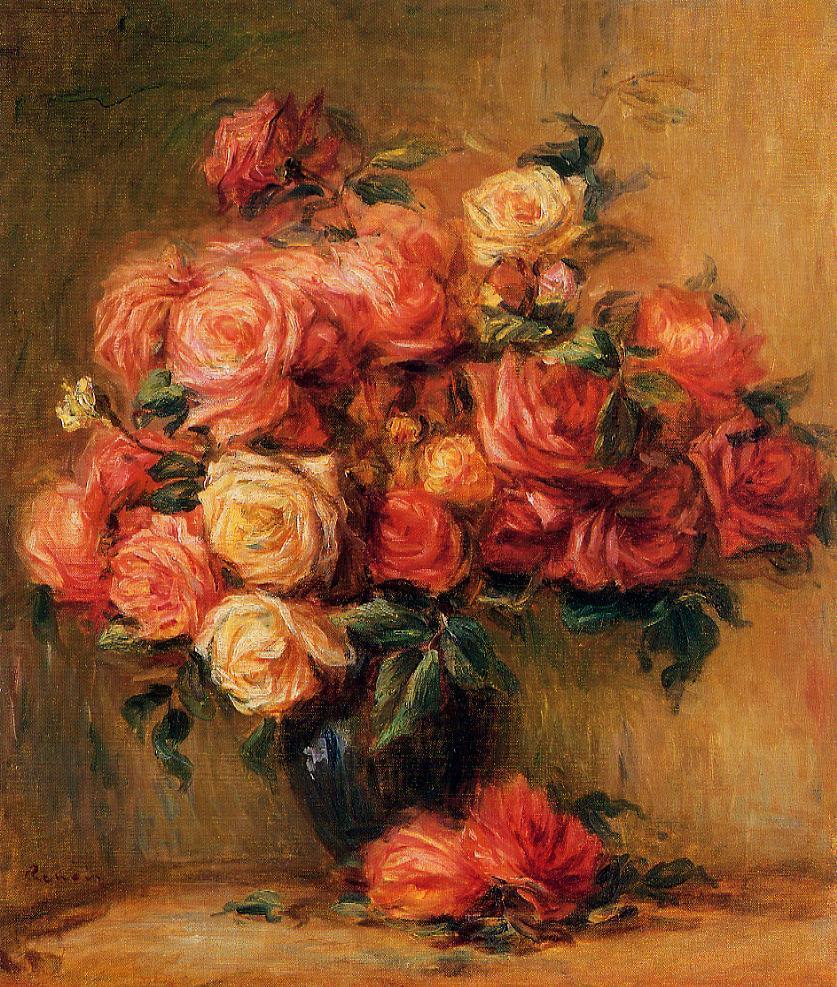This detailed oil pastel painting captures a vivid scene of approximately 20 roses in a black vase. The bouquet predominantly features pale pink and peach roses, interspersed with yellow, darker red, and white blooms, all displayed in varying stages of full blossom. Two roses have fallen near the bottom of the vase, accompanied by green leaves scattered around them.

The backdrop is a rich mix of golden hues with dark emerald green streaks on the left, providing a tangible depth and contrast that enhances the vibrancy of the flowers. The base, possibly a brown table or countertop, supports the vase and contributes to the earthy, muted palette. The painting deftly balances realism and painterly elements, with visible brushstrokes and swirling designs that add a textured, dynamic quality to the image. The highlights are executed using white, further accentuating the luminous quality of the roses and the subtle intricacies throughout the work.